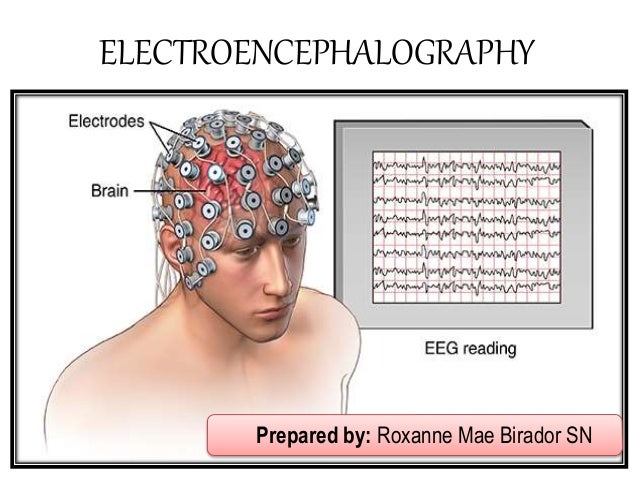This image, designed as a slide for a PowerPoint presentation, is a color illustration labeled "Electroencephalography" in bold black letters at the top. The centerpiece of the image is a detailed drawing of a young man, shirtless, with electrodes affixed to his head. These electrodes are depicted as silver cylindrical circles with black centers, and are clearly annotated with the word "electrodes" and arrows pointing to each. The man's brain is faintly visible in a pinkish hue, with the label "brain" pointing to it. To the right, a gray screen displaying fluctuating black lines is marked as an "EEG reading." In the bottom right corner, a light pink box with black text credits the preparation of the slide to Roxanne Mae Berador, S.N.